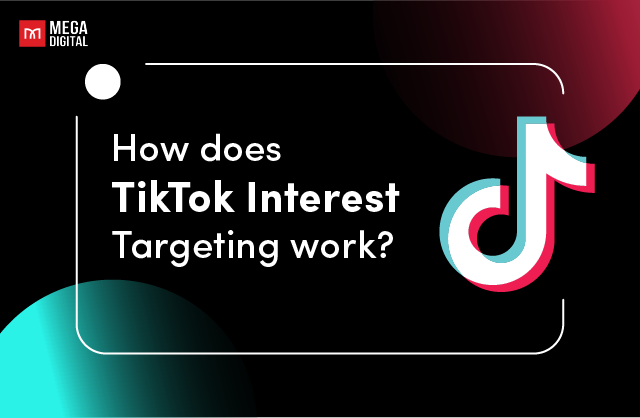This image is a promotional page for TikTok, featuring a visually striking design primarily in black, red, green, and white. The top left of the page has a green circular sphere, creating a focal point. Dominating the center of the page is a bold, white text in the middle of a red box that reads "MEGA DIGITAL." Directly below this headline, a white circle is encapsulated within a white rectangular border. Inside this box, another bold white text poses the question: "How does TikTok interest targeting work?"

To the right of this text, the iconic TikTok logo—comprised of blue, white, and red colors—stands out vividly. These elements contrast sharply against the background, which transitions from black in the top left and bottom right corners to red towards the top right and bottom left of the page. The overall design uses a minimalistic yet eye-catching color palette to draw attention to the key message and branding elements.